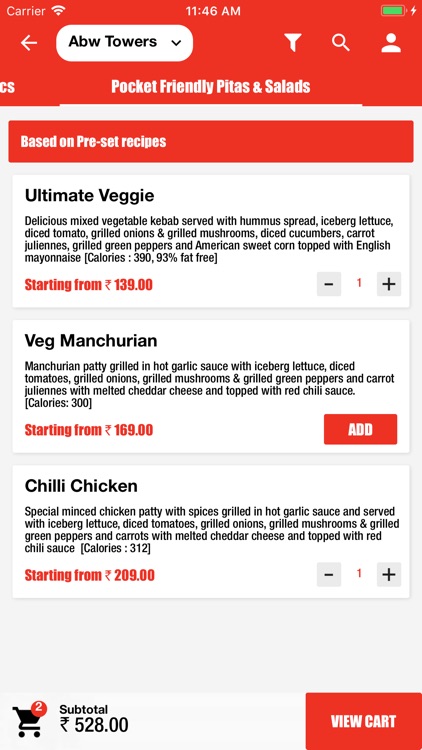A detailed caption: 

"The image showcases a digital takeout menu from Abu Towers, captured at 11:46 AM with a device battery at 96%. The menu highlights 'Pocket Friendly Pitas and Salads,' featuring a variety of preset recipes. Two options are ordered while another remains unselected. 

One ordered meal is the 'Ultimate Veggie,' a delectable mixed vegetable kebab served with hummus bread and an assortment of fresh vegetables including iceberg lettuce, diced tomatoes, grilled onions, grilled mushrooms, diced cucumbers, carrot juliennes, grilled green peppers, and American sweet corn, all topped with English mayonnaise. This dish offers 390 calories and prices start at 139 currency units.

The unselected item is a 'Manchurian Patty,' grilled in hot garlic sauce and accompanied by iceberg lettuce, diced tomatoes, grilled onions, grilled mushrooms, grilled green peppers, carrot juliennes, melted cheddar cheese, and finished with red chili sauce. This option starts at 169 currency units.

The second ordered item is 'Chili Chicken,' featuring a special minced chicken patty spiced and grilled in hot garlic sauce. It is served with the same array of vegetables and melted cheddar cheese, topped with red chili sauce. This dish has 312 calories with prices starting at 209 currency units.

The total cost of the two selected meals amounts to 528 currency units."